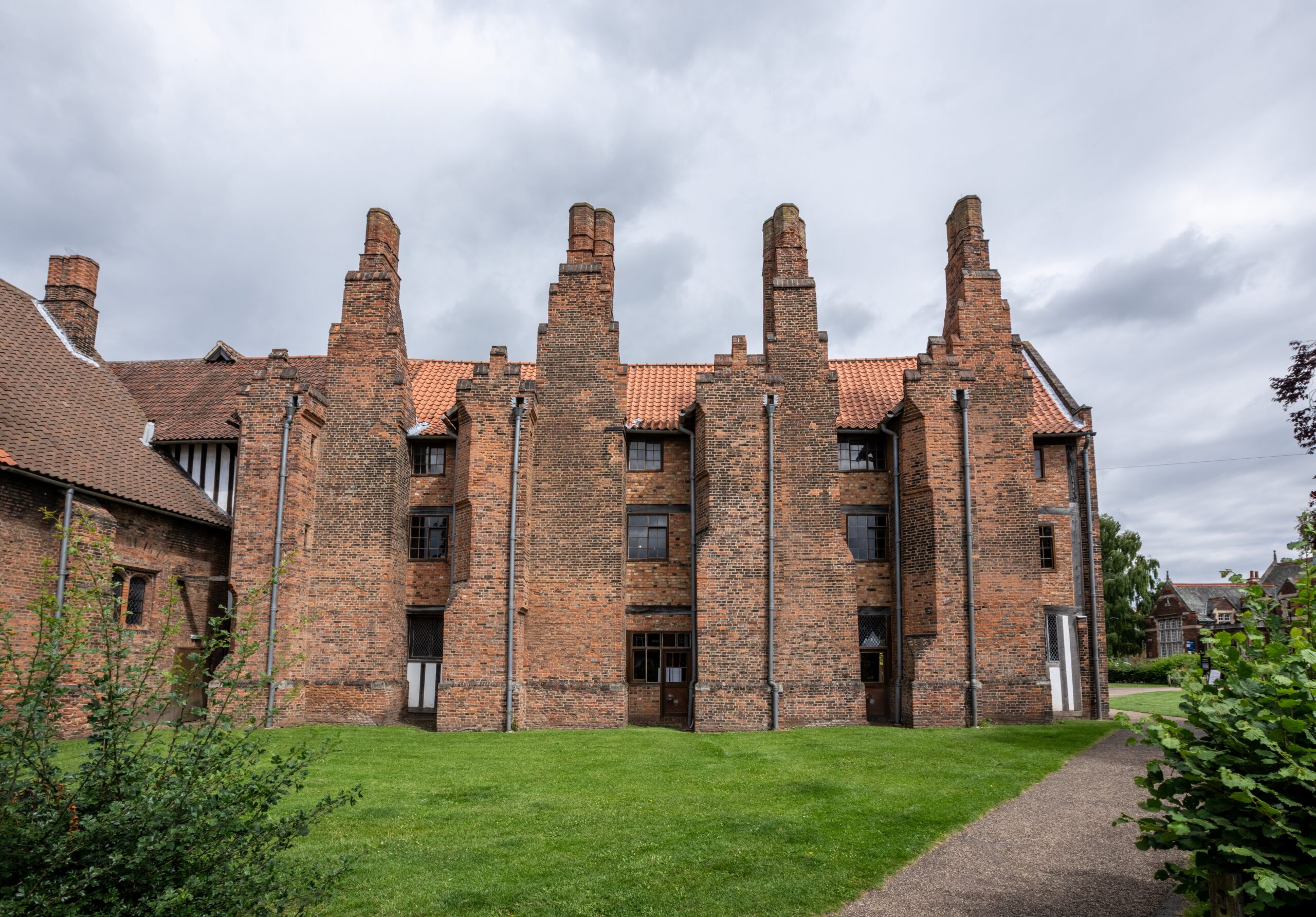The photograph showcases an English-style country mansion set against a backdrop of a well-maintained green lawn. The mansion is L-shaped, with the shorter arm of the L on the left-hand side of the image facing forward and the longer arm extending horizontally across the center. In front of the mansion, a neatly cut green lawn features a small bush in the lower left corner. On the right, a paved pathway runs diagonally from the bottom right to the center right, flanked by a large bush in the right corner. 

The building itself is constructed from weathered-looking sandstone bricks with various shades of tan and a rustic orange hue, suggesting age and exposure to the elements. The roof is two-toned, transitioning from a tan and orange color on the right-hand side to a deeper brown towards the back, indicating an older section of the structure. 

Striking pyramid-shaped pillars and large brick buttresses extend above the roofline. The mansion is three stories high, featuring numerous small windows situated between these four prominent brick buttresses. The left-hand side of the mansion is notably lower, resembling a single-story shed or garage area. 

In the far distance on the right-hand side, another English-style house can be seen, painted white with a tan roof. The sky above is gray and overcast, adding a moody atmosphere to the scene. This detailed architectural marvel, rich in historical and rustic elements, stands amidst a lush estate with similar period houses visible in the background.